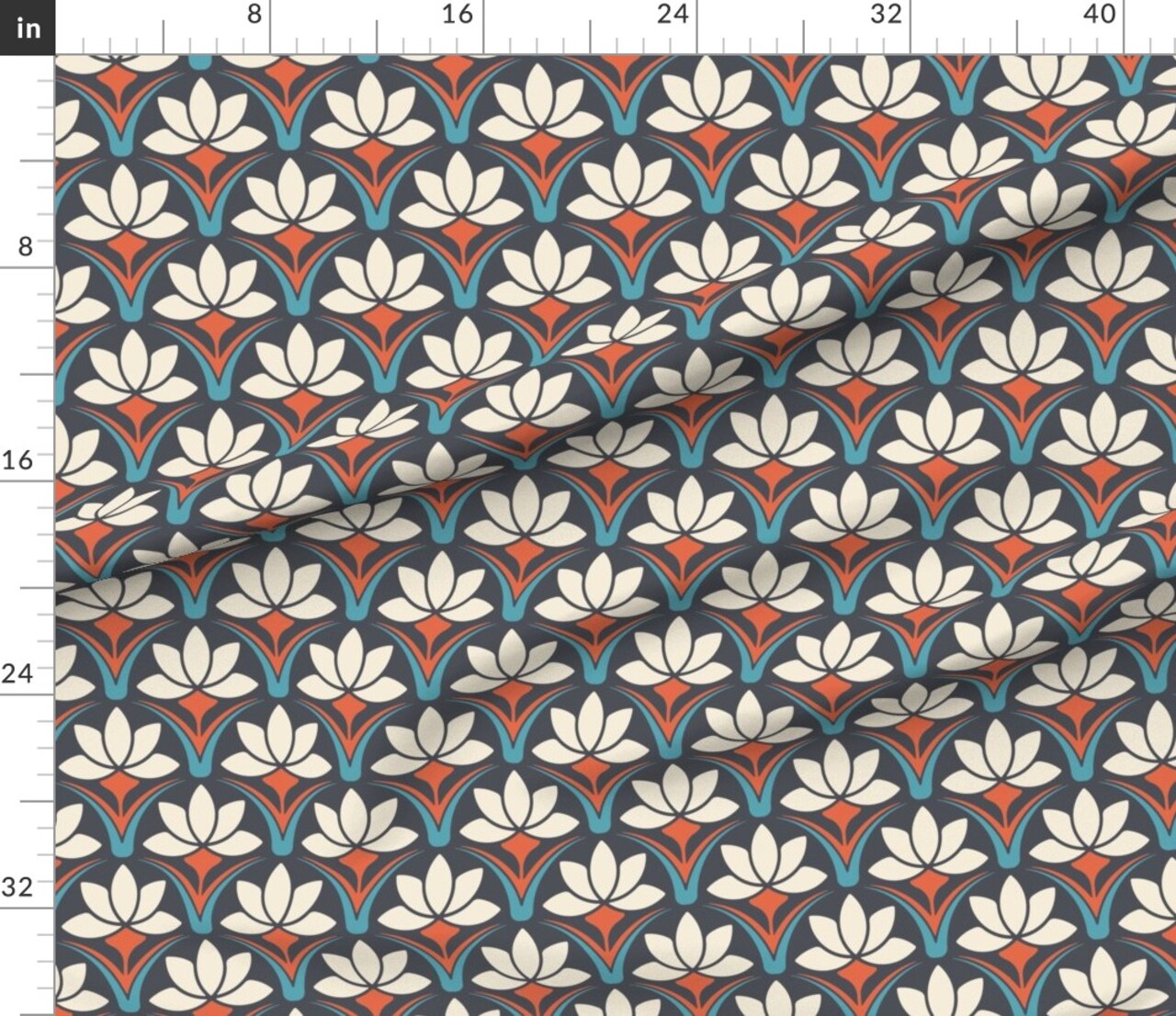The image features a slightly ruffled square piece of fabric, likely intended for sewing, displayed against a dark blue background with a detailed ruler along its top and left sides for precise measurement. This measuring guide, marked in inches, indicates lengths of up to 40 inches horizontally (X axis) and 32 inches vertically (Y axis). The fabric itself showcases a uniform pattern of five-petaled white lotus flowers, each seated atop a red stem. These stems connect to intricate designs comprising a red V and a blue V, creating an elegant repeated motif across the fabric. The overall dimensions of the fabric are roughly 43 inches wide and 35 inches tall, featuring measurements marked at intervals of 8, 16, 24, 32, and 40 inches.